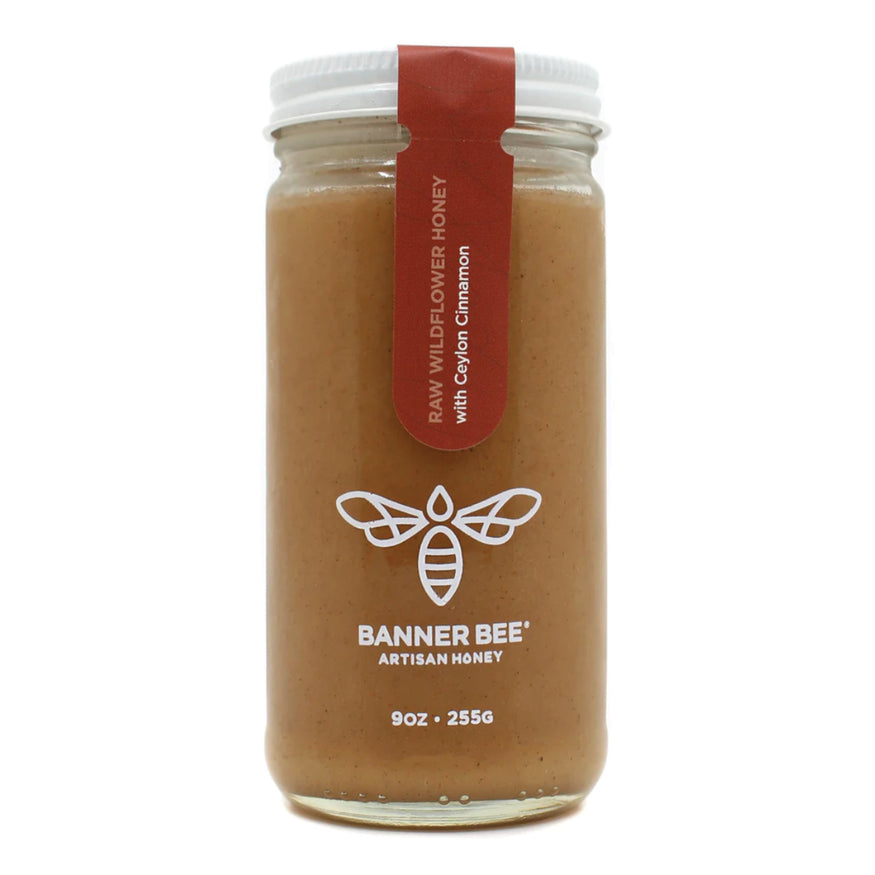The image showcases a 9-ounce (255 grams) glass jar of Banner Bee Artisanal Honey. The jar is adorned with a white metal cap featuring a dark red, tamper-proof seal that reads "Raw Wildflower Honey" in yellow text and "with Ceylon cinnamon" in white text. The honey inside is a light brown, thick, and viscous substance. The front of the jar prominently displays a custom bee logo above the text "Banner Bee Artisanal Honey," with "9 ounces, 255 g" written underneath, separated by a small white dot. The entire scene is set against a pristine white background, emphasizing the jar as the sole focus of the image.